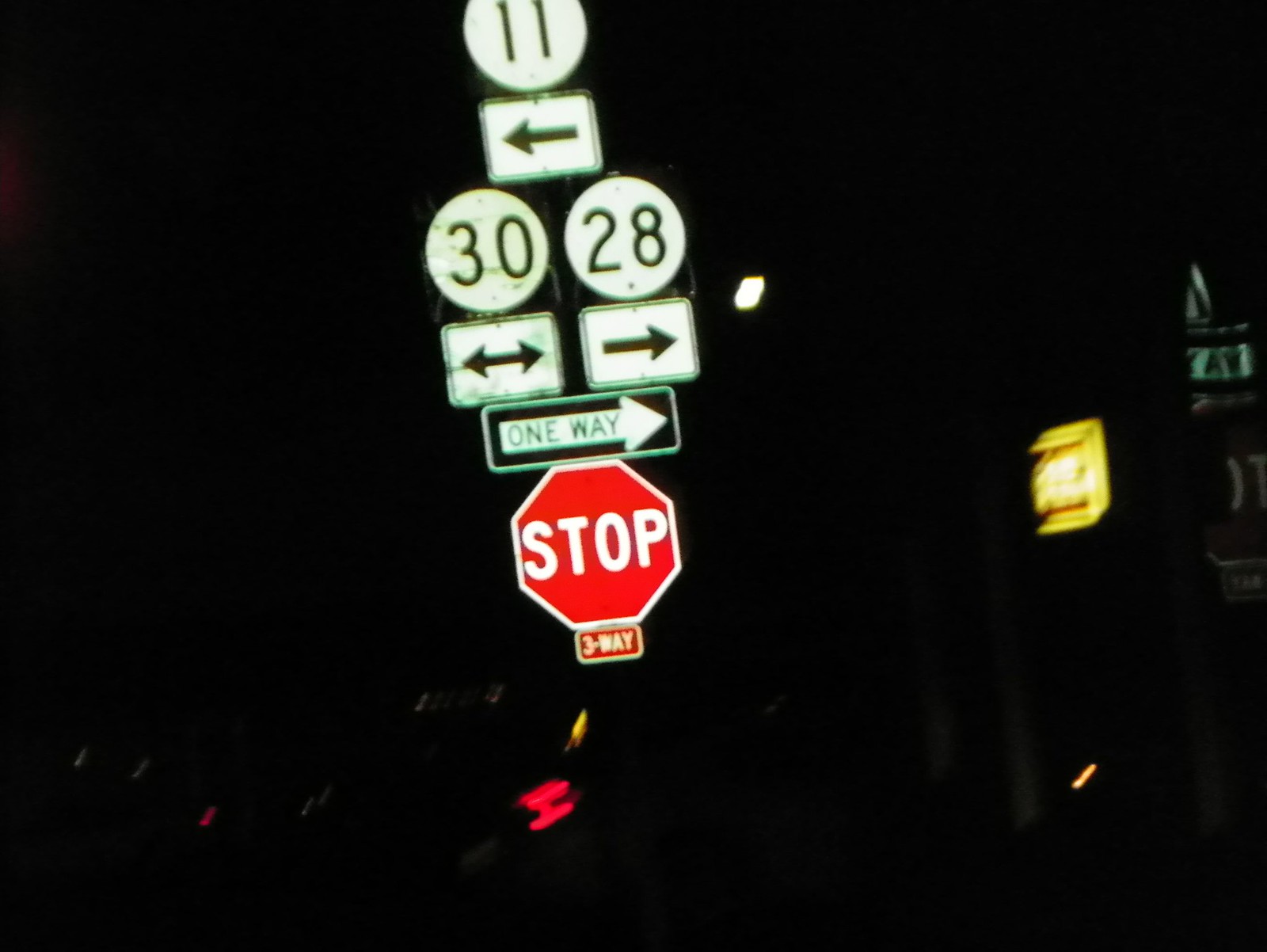Captured during a nighttime drive, this photograph showcases a collection of road signs illuminated against a dark backdrop. Central to the image is a vertical array of signage. At the top, a white circular sign bears the number "11" in black. Directly below, a rectangular white sign features a left-pointing black arrow. Next, two adjacent circular signs display the numbers "30" and "28" respectively. Beneath these, two rectangular signs show directional arrows: one sign points both left and right, while the other solely points right. Further down, a black one-way sign with a white arrow is present. Below it, a brightly lit red stop sign includes a small "three-way" label underneath. The scene is enhanced by the presence of blurred red and yellow traffic lights at the bottom of the frame, capturing the motion of passing vehicles and adding a sense of dynamic movement to the still image.